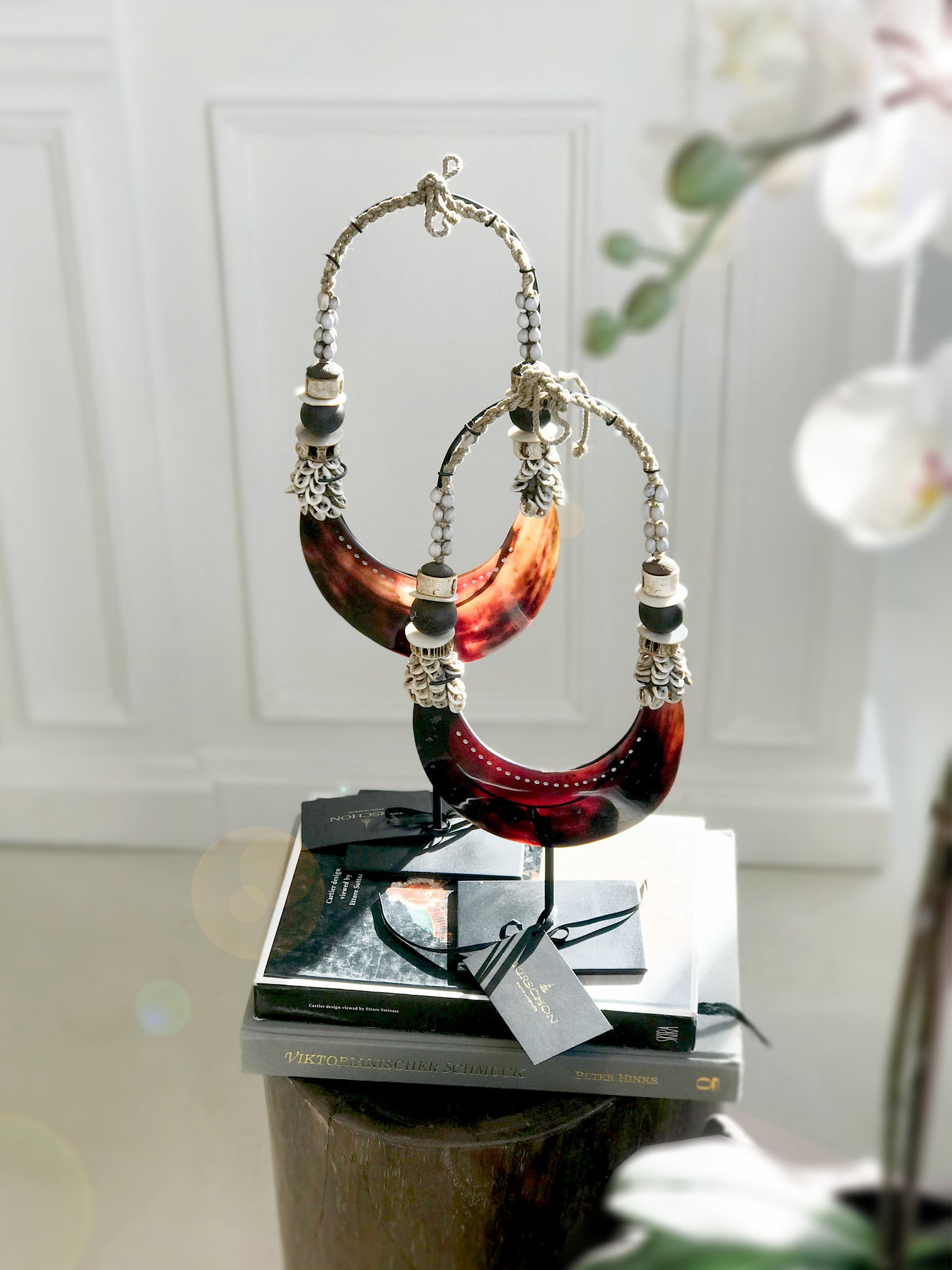The image features a sophisticated indoor display showcasing unique jewelry pieces set against a detailed white wall with crown molding and square accents. In the background, a plant with white petals and green leaves can be seen, adding a touch of nature to the scene. The floor is a neutral gray.

At the center, there is a smooth brown wooden stool or log that serves as a display table. On top of this wooden stand sit two books - one gray with gold letters and one black. Additionally, several company cards are visible on the books, suggesting the jewelry might be from a specific brand.

The main focus is the jewelry, elegantly arranged on two black stands. These stands hold jewelry pieces that feature intricate silver bands connected to colorful glass components. One jewelry piece at the back integrates a semi-translucent tortoiseshell pattern in a maroon and yellow color scheme, shaped like a gemstone. The piece in the front showcases a design with dark red glass, adorned with white dots and silver scale-like elements. Both pieces exude a blend of artistic craftsmanship and aesthetic appeal, making the display both eye-catching and refined.